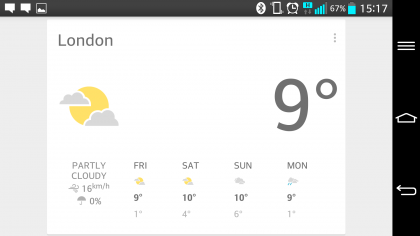The image displays a mobile phone screen in horizontal orientation showing weather information. The top header has a dark grey background with several icons lined up. On the top left, there are two white chat box icons followed by a thumbnail image icon. Next to these is a Bluetooth icon, resembling an angular bee with two lines extending from the back at 45-degree angles, and a small rectangle with small lines around its top left and bottom right corners. This is followed by a classic alarm clock icon. Continuing to the right, there are two grey arrows with a blue box labeled 'H' above them. Further to the right are the mobile signal bars, which are blue and increase in height from left to right, except the tallest bar which is grey. Adjacent to these bars, the text '67%' is displayed, alongside a battery icon showing the same percentage. Next to the battery icon, the time '15:17' is displayed.

On the right edge of the screen, a vertical black bar contains three icons: three horizontal white lines at the top, a squished home icon in the center, and a white arrow that curls up and points left at the bottom.

The main portion of the screen has a light grey background with a prominent white rectangle containing the weather information. At the top left within this rectangle, the location 'London' is displayed. Beneath this, there is an icon of the sun partially obscured by two grey clouds with a temperature reading of '9°C' to the right. Below the icon, the phrase 'Partly Cloudy' is displayed. The bottom section of the rectangle shows a four-day forecast with the days listed as Friday, Saturday, Sunday, and Monday, with respective temperatures of 9°C, 10°C, 10°C, and 9°C.